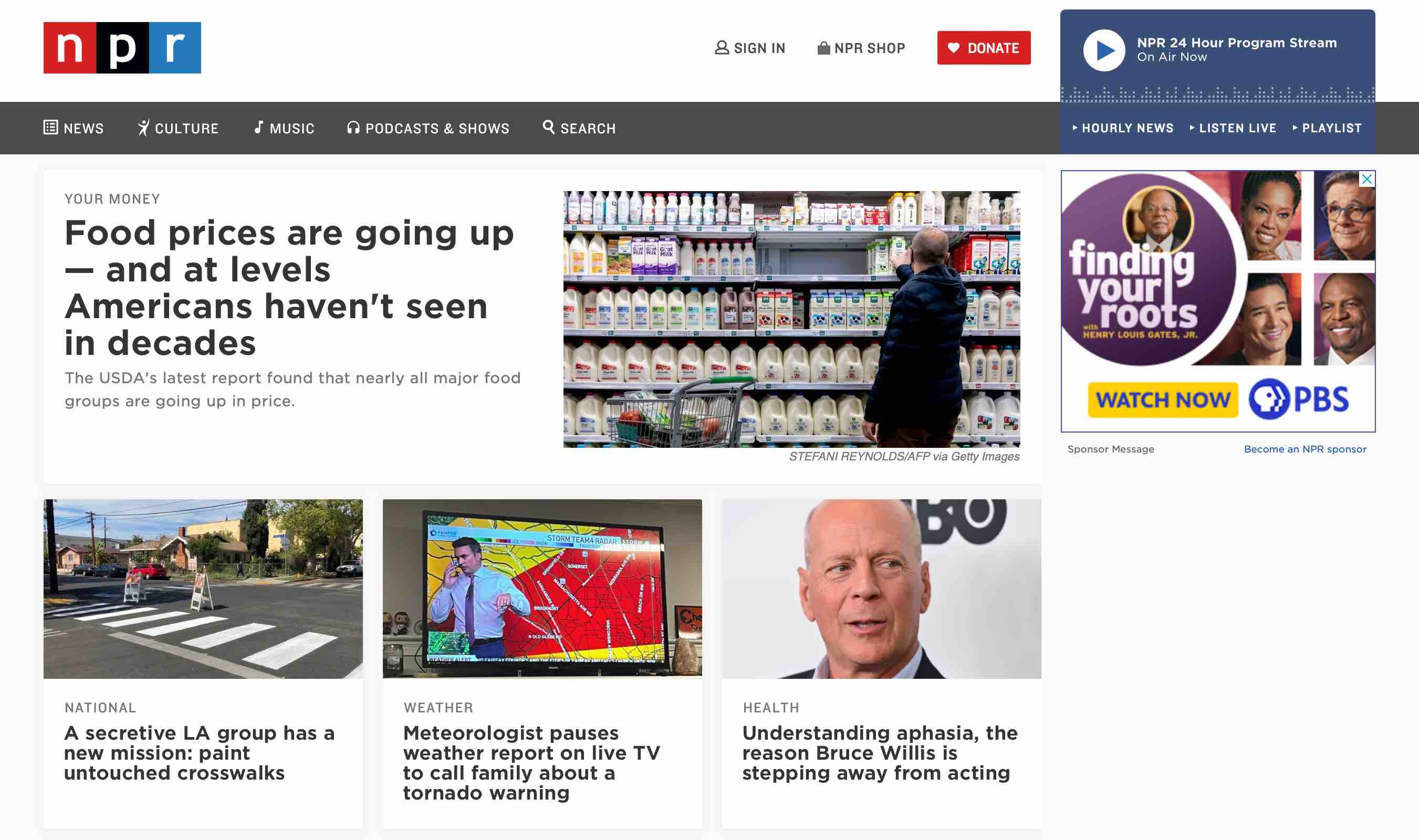The image features a white background. In the top left corner, there are three colorful squares—red, black, and blue—each containing the letters "NPR." Next to these boxes, there are options labeled "Sign In," "NPR Shop," and a prominent red "Donate" button. Adjacent to these elements, there's a blue box with a white circle containing a blue arrow pointing to the right, labeled "NPR 24-Hour Program Stream," along with "On Air Now." This section also includes options such as "Hourly News," "Listen Live," and "Playlist."

Below this, there's a white box with text that states: "Your Money. Food prices are going up at levels Americans haven't seen in decades." To the right of this text, there is an image depicting a man in a grocery store.

On the far right, there is another box featuring four smaller squares, each containing a different person's picture, along with a larger purple circle that includes an image and the text "Finding Your Roots." Below this, it says "Watch now on PBS," accompanied by some smaller blueprint text.

At the bottom of the image, there are three smaller pictures with captions: 
1. "A Secretive LA Group has a New Mission: Paint Untouched Crosswalks."
2. "Meteorologist Pauses Weather Report on Live TV to Call Family About a Tornado Warning."
3. "Understanding Aphasia: The Reason Bruce Willis is Stepping Away from Acting."